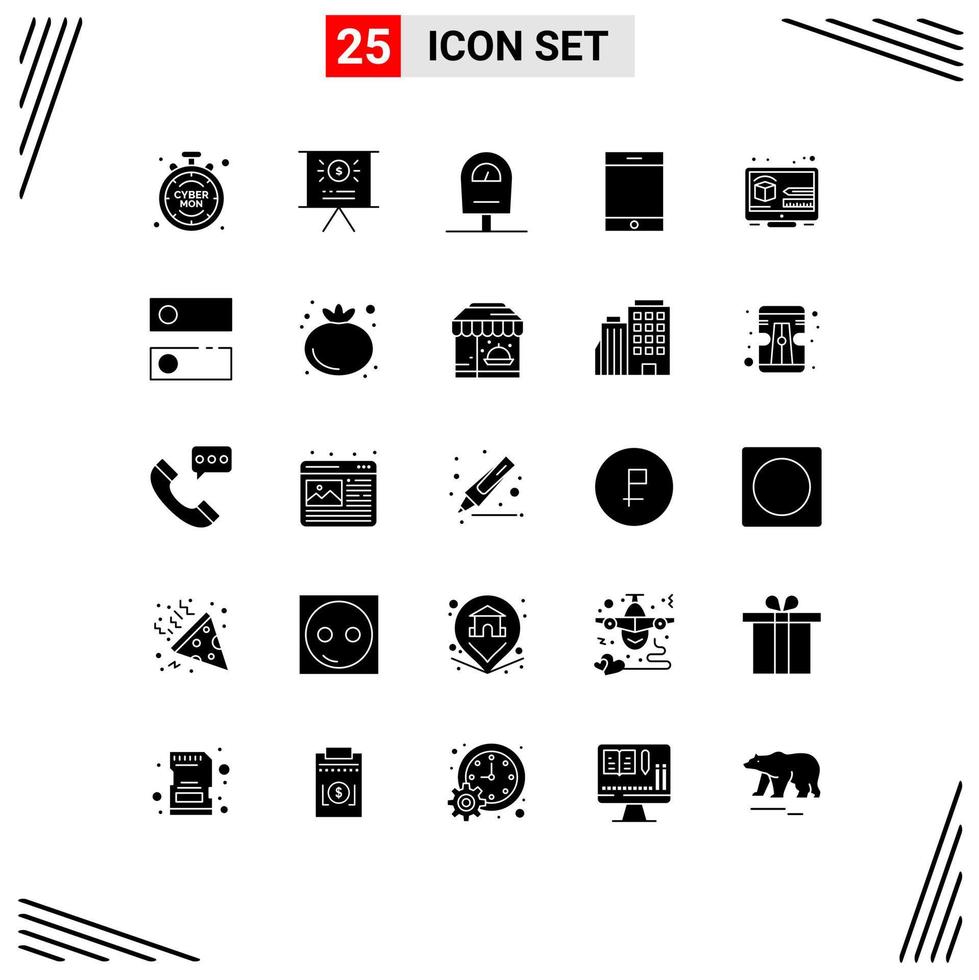The image is a detailed icon set displayed on a white background, with the title "25 Icon Set" prominently featured above. The number '25' is printed in white on a red background, while "Icon Set" is rendered in black on a gray background. The icons are meticulously arranged in a 5x5 grid, with five icons per row and five rows in total. Each corner of the image is accentuated with diagonal lines, framing the entire illustration.

In the first row (left to right): 
1. A stopwatch labeled "Cyber M.O.N."
2. A television displaying a money symbol.
3. A parking meter.
4. A dishwasher.
5. A computer screen.

In the second row (left to right):
1. Two rectangles stacked vertically; the top rectangle is black with a white-outlined circle, and the bottom rectangle is white with a black-filled circle.
2. A black tomato.
3. A storefront with an awning and a serving platter.
4. Two high-rise buildings.
5. A football field.

In the third row (left to right): 
1. A telephone with a speech bubble.
2. A PowerPoint slide.
3. A black ink pen pointing down and to the left.
4. A black circle with a square flag intersected by a horizontal white line.
5. A black square with a white-outlined circle inside.

In the fourth row (left to right):
1. A piece of pizza with squiggly lines, oriented down and to the right.
2. A black square with a white-outlined smiley face.
3. A location pin with a building inside.
4. A black and white airplane facing the viewer.
5. A black and white gift box.

In the fifth row (left to right):
1. An SD card drawn in black and white.
2. A black square featuring a dollar sign.
3. A clock set to nine o'clock with a gear wheel partially obscuring the lower left.
4. A computer monitor with a book and pencil icon.
5. A black bear facing left.

Overall, the detailed illustration effectively presents 25 distinct black and white icons, all neatly organized and clearly defined against the clean white backdrop.